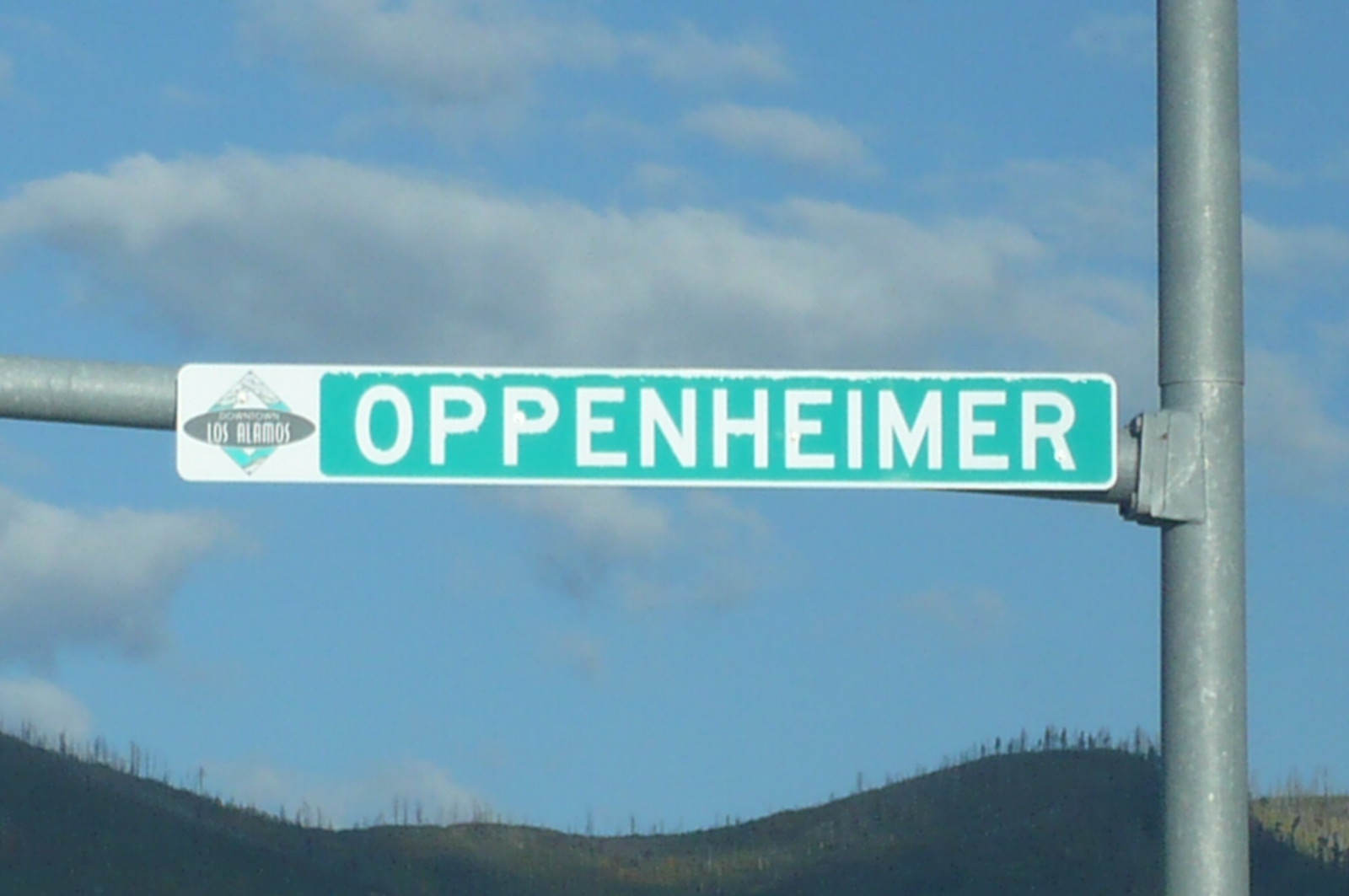The image depicts a street sign on a tall, metal pole featuring the name "Oppenheimer" in white letters on a green background. The sign is horizontally affixed to a curved lateral arm extending from the vertical post, which continues out of the frame both to the left and at the top and bottom. On the left side of the sign, there's a turquoise and dark gray logo with an oval inside a diamond shape and the text "Los Alamos." The background showcases rolling hills with sparse vegetation and patches of dirt or sand. Above the hills, a bright blue sky is filled with evenly spaced, fluffy white clouds, creating a serene and expansive atmosphere.